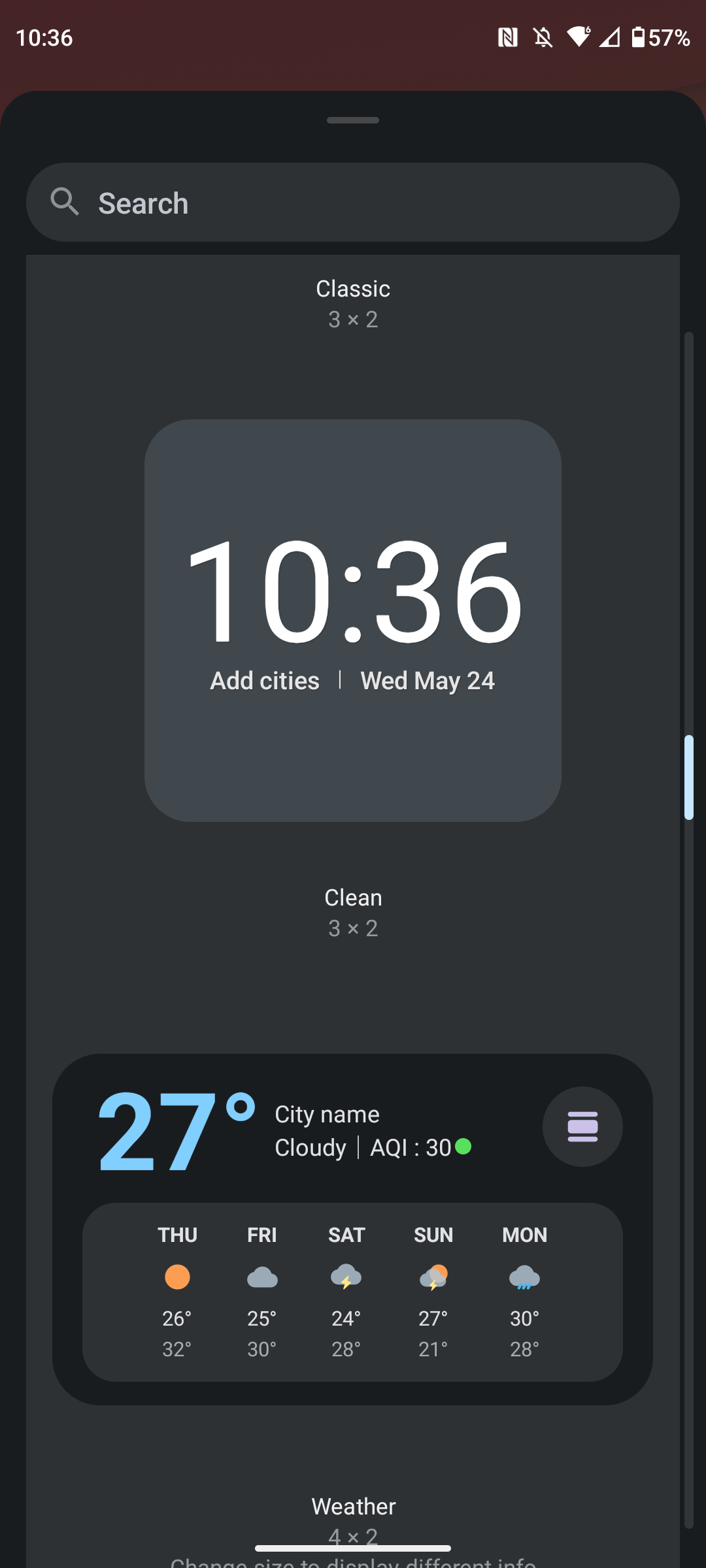This image is a screenshot captured on a cell phone with a portrait orientation, approximately two to three times taller than it is wide, and rectangular in shape. At the top of the screenshot, there is a reddish-brown horizontal border containing white text and icons. On the left side, the number "1036" is displayed. Moving rightwards, there is an assortment of icons: an 'N' icon, a bell with a line through it indicating silent mode, a full wifi signal icon, a cell service meter that is less than 50% full, and a battery icon showing 57% with a vertical white meter.

Below this border, a noticeable black box with a similar horizontal tab on top is present. This is followed by a gray search bar with white text. The background of the screenshot is gray and also in portrait orientation, featuring centered white text that reads "Classic 3x2." 

Further down, there is a gray box with rounded edges displaying "1036" in white text. Below this, in smaller white text, it says "Add Cities" followed by "Wednesday, May 24th."

Towards the bottom of the screenshot, the text "Clean 3x2" is visible, followed by a black landscape box. Within this box, light blue numbering shows "27 degrees," accompanied by text that reads "City Name, Cloudy." Below this bit of weather information, there is a small box with the weather forecast spanning from Thursday to Monday.